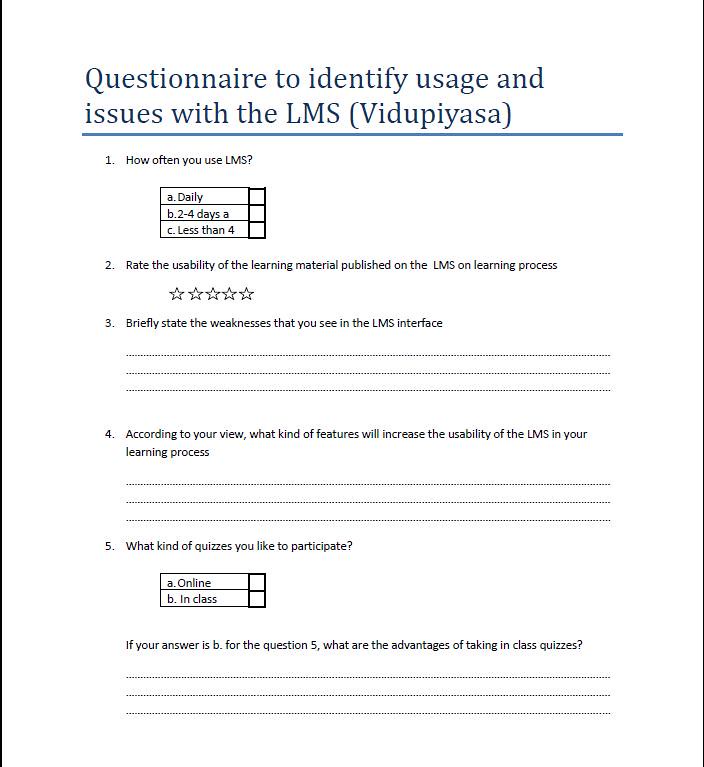The image depicts a white paper questionnaire titled "Questionnaire to Identify Usage and Issues with the LMS" in blue text, intended to gather feedback on a Learning Management System (LMS). Beneath the title, the name "Vidu Paisa" appears in blue with an underline. The questionnaire consists of five questions numbered sequentially on the left side. Each question is in blue text:

1. **How often do you use LMS?** 
    - Options: A. Daily B. Two to four days C. Less than four days
    
2. **Rate the usability of the learning material published on the LMS learning process:** 
    - Five-star rating system provided
    
3. **Briefly state the weaknesses that you see in the LMS interface:**
    - Open-ended with three lines for the response
    
4. **According to your view, what kind of features will increase the usability of LMS in your learning process?**
    - Open-ended with three lines for the response
    
5. **What kind of quizzes would you like to participate in?**
    - Options: A. Online B. In class
    - Follow-up: If you answered B, what are the advantages of taking in-class quizzes?
        - Open-ended with three lines for the response